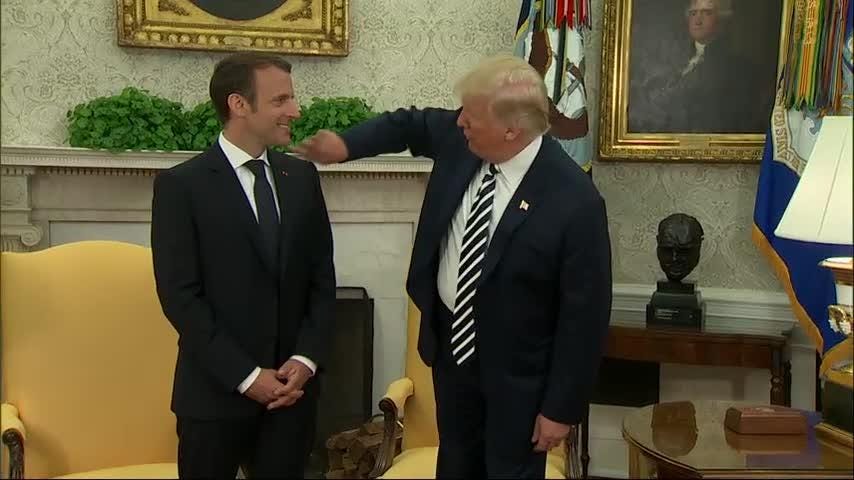This detailed photograph captures a moment inside the Oval Office in the White House, featuring then-President Donald Trump and French President Emmanuel Macron. The two leaders stand side by side, with Trump pointing at Macron, who responds with a smile while looking sideways at Trump. Donald Trump is dressed in a black suit, a white shirt, and a black and white striped tie, with an American flag pin on his lapel. Macron mirrors Trump’s attire with a black suit and white shirt but opts for a solid black tie and wears a pin on his lapel as well, though its details are not clearly identifiable.

In the rich backdrop, the presidential setting of the Oval Office is brought to life with several notable elements. Behind the pair, prominently displayed, is a gold-framed oil painting of Thomas Jefferson, which hangs on the wallpapered wall above the fireplace adorned with greenery. Adjacent to it, on a side wooden table, sits a dark-colored bust. Another portrait, that of George Washington, can be partially spotted beneath the top corners of the fireplace. Two yellow armchairs with wooden arms flank the room, contributing to the stately decor. Additional elements such as the United States flag, a lamp on a side table, and a brown table with a glass top enrich the setting, framing this significant diplomatic interaction within the iconic Oval Office.